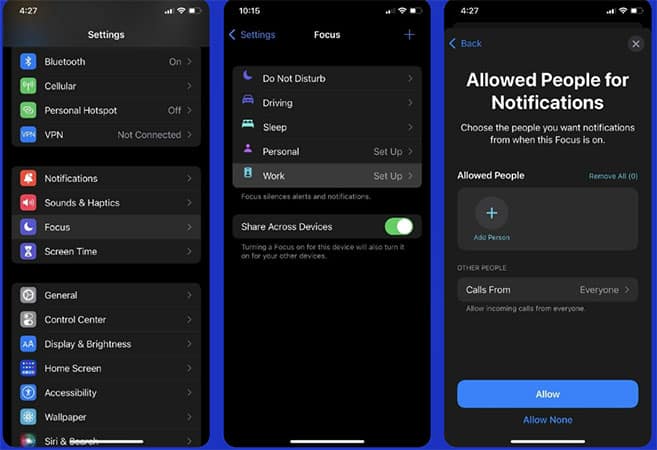**Caption:**

The collage features three images displayed side-by-side. The image on the left shows the time as 4:27 and lists several device settings. Each setting is accompanied by an icon on the left side of the list. From top to bottom, the settings include: 

- Bluetooth (with the status indicated as 'On')
- Cellular
- Personal Hotspot (with the status indicated as 'Off')
- VPN (with the status 'Not Connected')
- Notifications
- Sound & Haptics
- Focus
- Screen Time
- General
- Control Center
- Display & Brightness
- Home Screen
- Accessibility
- Wallpaper
- Siri & Search

The middle image highlights the 'Focus' settings section. At the top, it shows a labeled section for 'Do Not Disturb,' 'Driving,' 'Sleep,' 'Personal Setup,' and 'Work Setup.' Below this list, there is an option labeled 'Share Across Devices' with a toggle switch to the right, which is in the 'enabled' position and highlighted in green color.

The image on the right provides a closer look at the 'Focus' settings, emphasizing the detailed options available under the 'Do Not Disturb,' 'Driving,' 'Sleep,' 'Personal Setup,' and 'Work Setup' categories. The 'Share Across Devices' feature is similarly displayed, with its toggle switch turned on, denoted by a green hue.